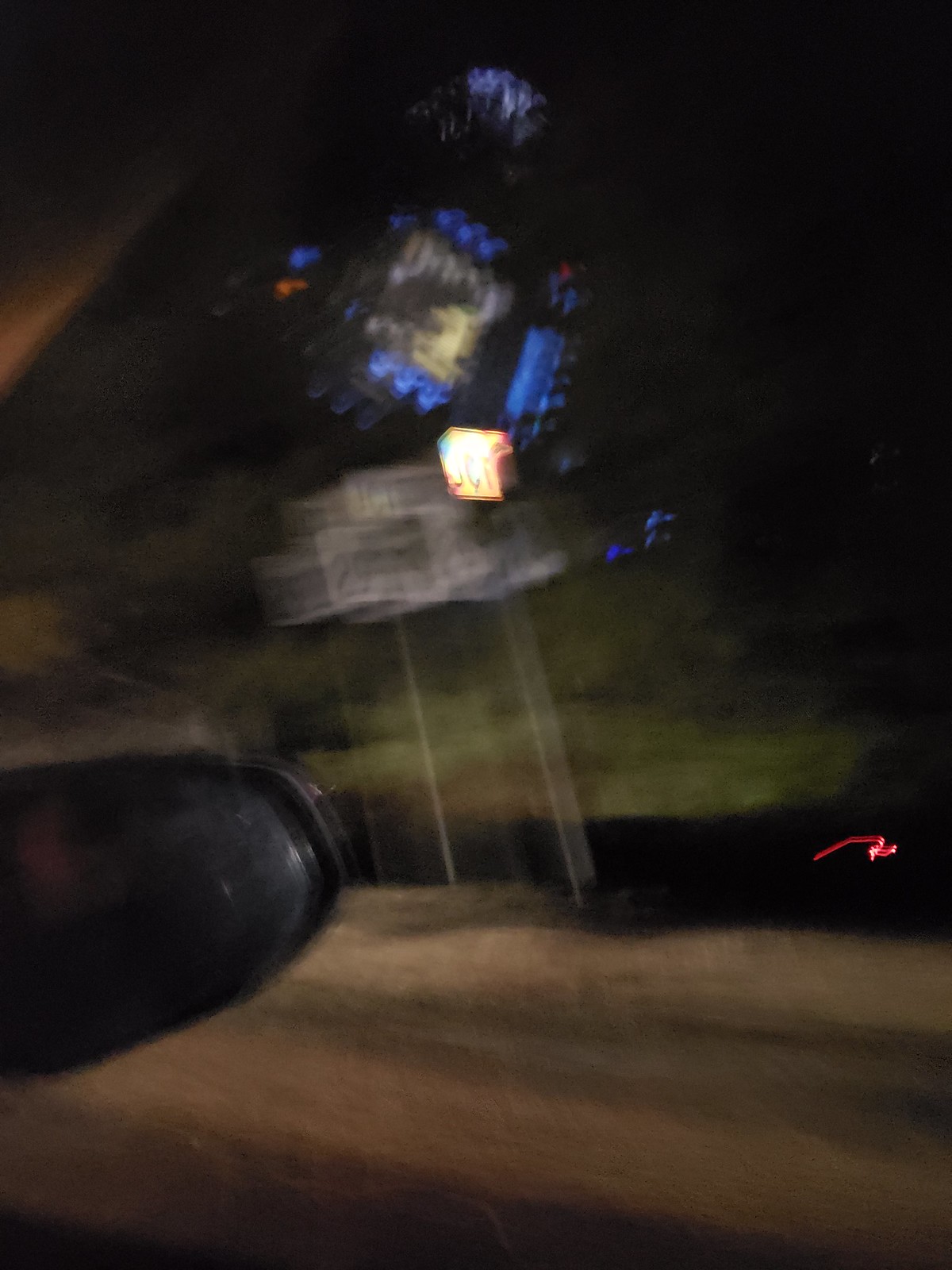This photograph, evidently captured from the passenger seat of a moving vehicle, features distinctive elements that illustrate a reflective, fast-paced environment. The left side of the image includes a visible side view mirror, reinforcing the view from within the car. The window appears rolled up, contributing to harsh reflections originating from inside the vehicle, possibly off of a white panel with blue and orange lights, which might be part of the center console. 

The scene outside the window is markedly blurry, suggesting the car's motion. The roadside features a cluster of indistinct signs, likely displaying numbers which are only partially decipherable, possibly including digits like "2" and "9." The background hints at a mix of trees and grass, adding to the unclear yet dynamic portrayal of a journey in progress.